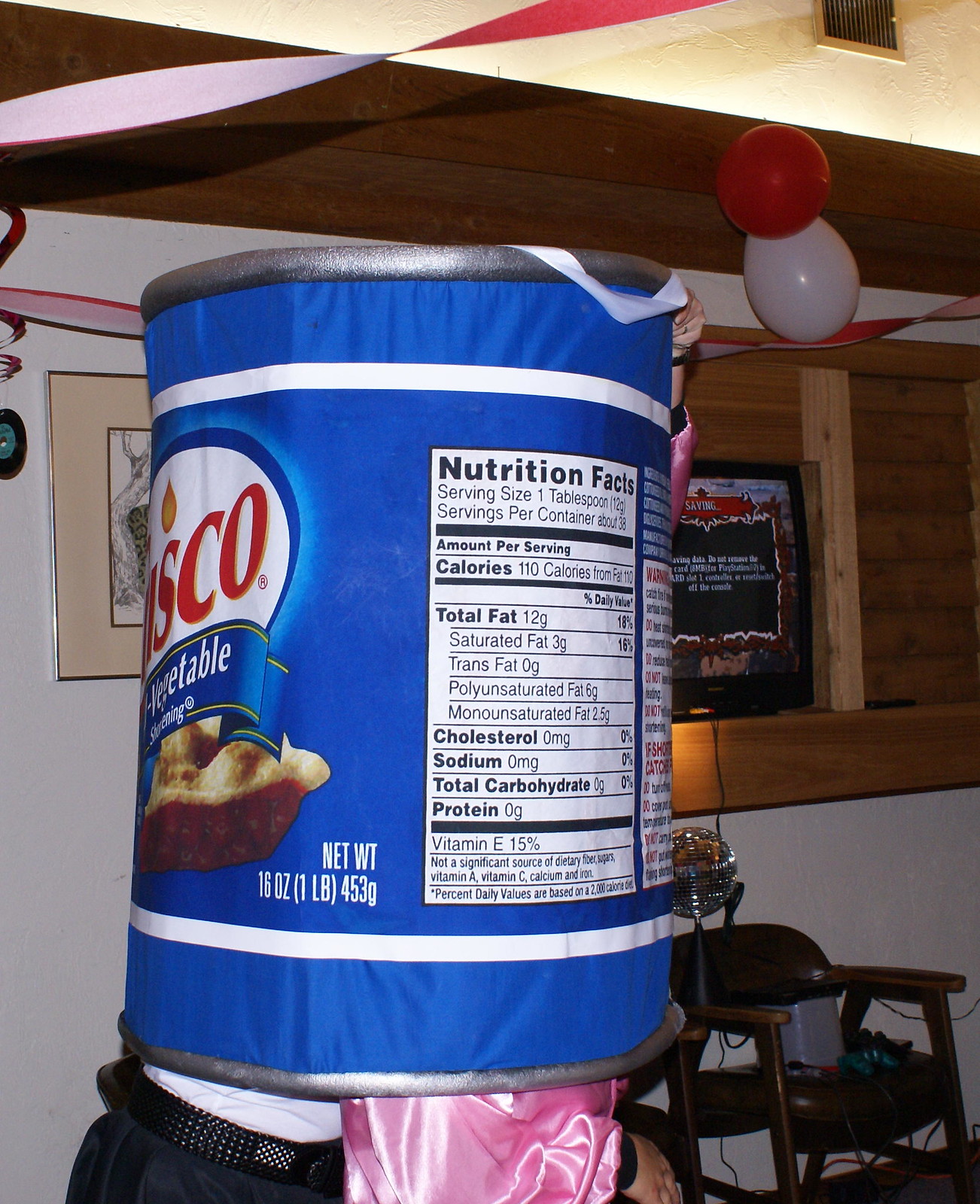In the center of this vertically-oriented image, there is a detailed imitation of a Crisco can, which appears to be a Halloween costume. The costume is a cylindrical, fabric reproduction of a medium blue Crisco vegetable shortening can, complete with realistic wrinkles and texture. The can has two horizontal white stripes at the top and bottom, with the word "Crisco" visible on the left. It features a nutrition label with detailed information including calories, total fat, saturated fat, cholesterol, and sodium in black and white. Additionally, it has a silver rim at both the top and bottom.

Emerging from the bottom of the can, you can see a man’s waist, clad in a black belt, a white shirt, and dark-colored dress pants, confirming it is a worn costume. Furthermore, a hand, possibly wearing a pink puffy shirt, is seen protruding, suggesting another participant or a prop accessory is involved.

The background reveals it is set in a basement-like space, indicative of a party environment. Red and white balloons are floating, and there are additional details such as a chair with a disco ball on a pillar, picture frames on the wall, and a cut-out space resembling a TV area. The setting is further characterized by wooden paneling and various other household items, contributing to the lively, festive atmosphere of a basement party.